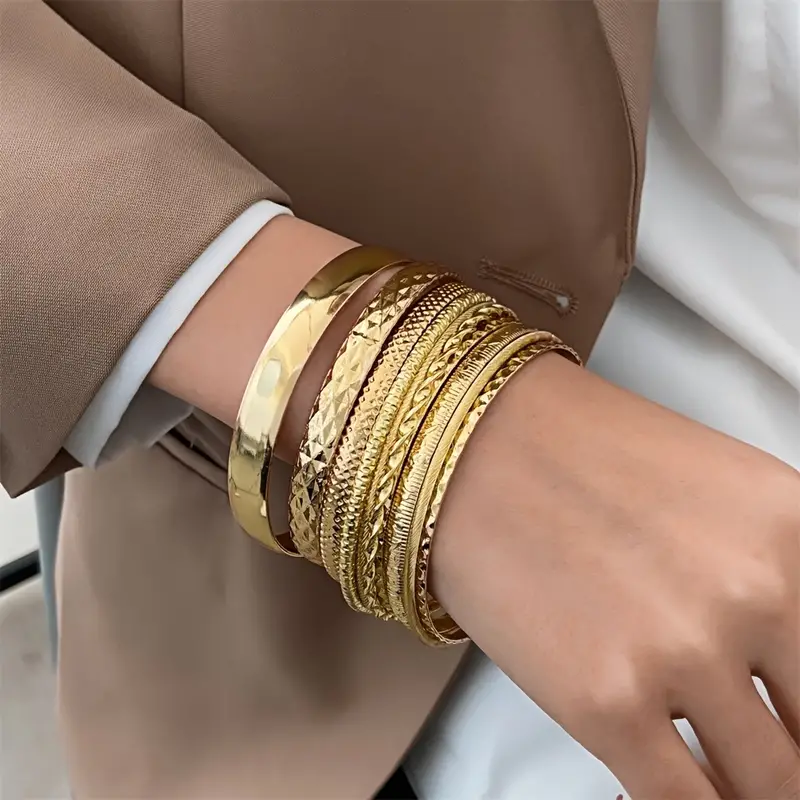This image captures a close-up of a woman's right hand and wrist, dressed in a light chocolate brown blazer with a white blouse underneath. The arm extends diagonally from the upper left corner towards the lower right corner, with parts of her little finger, ring finger, and middle finger slightly visible at the bottom right. She is adorned with at least seven or eight intricately designed gold bangles, varying in thickness and patterns. The two bangles closest to her wrist are notably thicker, while those nearer to her hand are thinner and closely spaced. The gold bangles feature unique beveling and ornate designs. The blazer and shirt sleeves are visible around her arm, enhancing the elegant presentation of her jewelry.